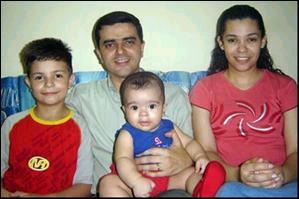This photograph captures a close-knit family of four sitting together on a blue couch. In the center sits the father, a man with short black hair, dressed in a white button-down shirt, holding a small baby, approximately six months old, who is wearing a blue t-shirt, red shorts, and matching red booties. To the father's left is the older son, a young boy with short hair, dressed in a red and white t-shirt with a yellow collar. On the right side of the couch is the mother, a woman with long black hair and tan skin, wearing a red t-shirt adorned with a distinctive swirly five-part white design. The family appears comfortable and connected, with the mother's hands folded gently in her lap.